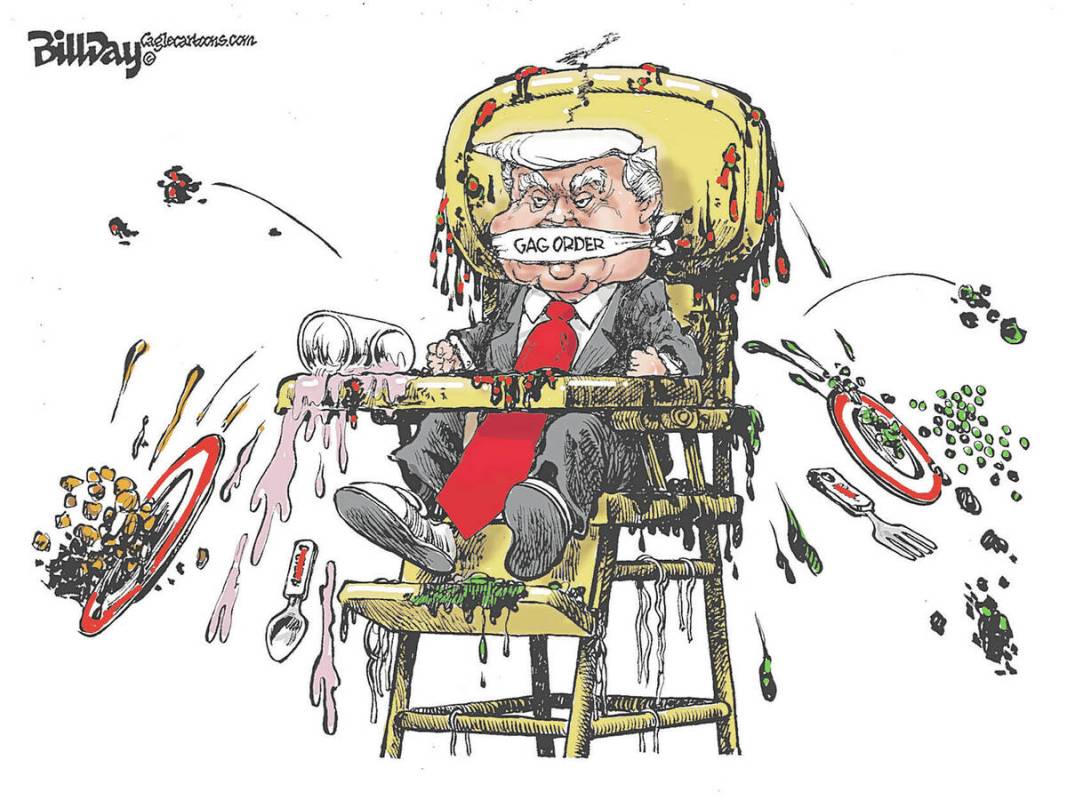This comical and detailed political cartoon by Bill Day, visible on the top left with his name and EagleCartoons.com, centers around a caricature of Donald Trump depicted as a frustrated toddler in a yellow high chair, spilling food everywhere. Trump's characteristic white hair is intact, and he is humorously restrained by a white bandana across his mouth that reads "Gag Order." The high chair is covered in various types of food, with a pink liquid spilling off to the left from a fallen glass, red and black food scattered on the top, and green and black food near the bottom. Two children's spoons with red lines are seen falling off each side of the high chair. In front of the high chair are two plates, one to the left with golden food exploding from it and another on the top right with green peas raining down. The cartoon vividly captures the essence of a temper tantrum, suggesting Trump's frustration and anger over the gag order.